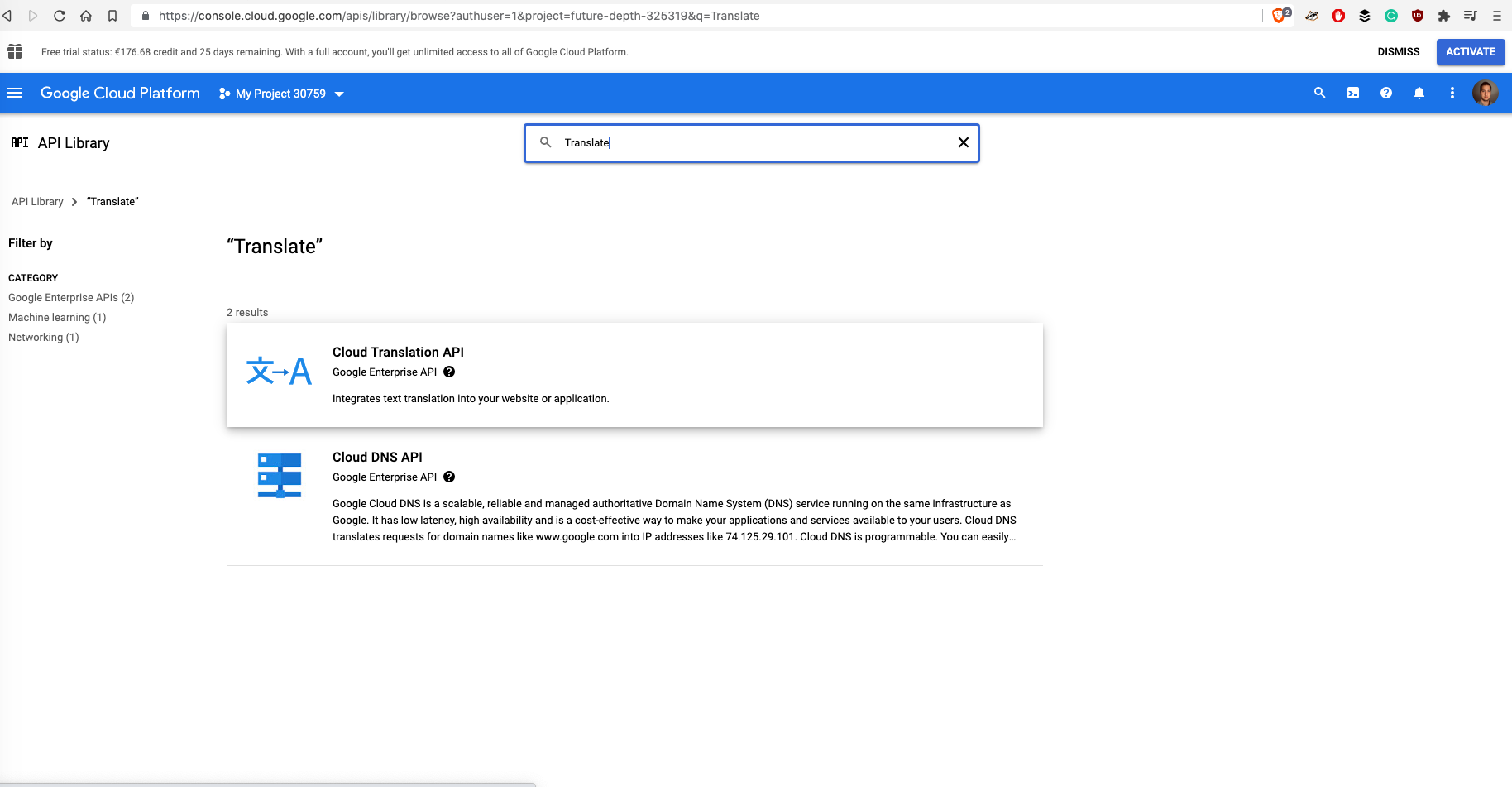Screenshot of a Google Cloud Console webpage displaying various features and information.

At the top of the screen, the URL reads "https://console.cloud.google.com/". Below the URL, there's a notification bar indicating a "Free trial status" with a balance of £176.68 credit and 25 days remaining. The notification mentions that, with a full account, you'll get unlimited access to all of Google Cloud Platform.

A prominent blue rectangle banner labeled "Google Cloud Platform" spans the entire width of the screen. On the left side of this banner, it shows the project name "My Project 30759". On the far right of the banner, there are several icons, including a profile picture of a man.

Further down on the page, there are sections for different APIs including:
- "API Library" 
- "Translation"
- "Cloud Translation API"
- "Cloud DNS API"
- "Google Enterprise API"

Each section has a brief description underneath its title.

In the center of the page, there is a white box bordered by a blue line, also in the shape of a rectangle, with the word "Translate" prominently displayed inside it. The overall layout showcases various Google Cloud Platform services and features accessible from the console.